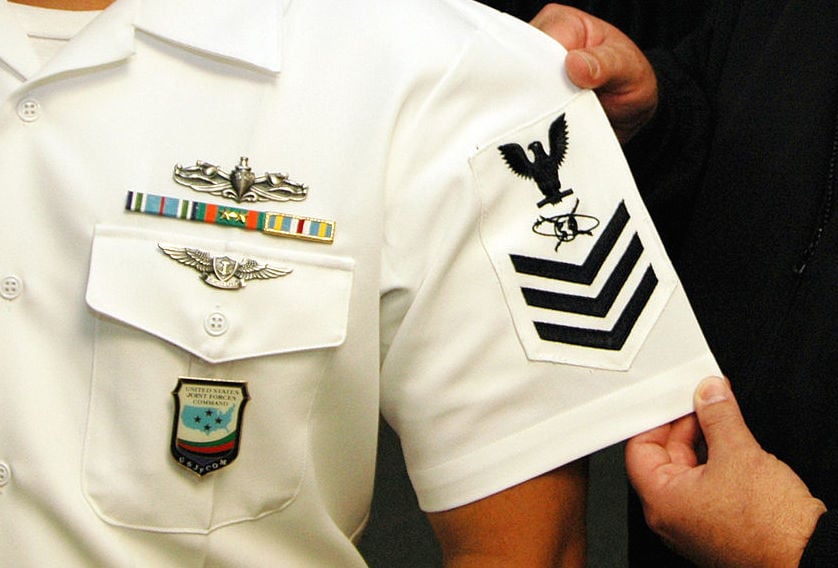This image captures a detailed close-up of a sailor's left arm and upper chest, showcasing his recent promotion. Wearing crisp white attire, the sailor prominently displays the rank insignia of a Chief Petty Officer with three downward arrows or chevrons and an eagle, visible on his sleeve. His chest is adorned with three ribbons and two distinctive badges: the insignia for submarine service and aviator wings, indicating his dual qualifications. There is also an additional mysterious medal, potentially symbolizing another notable achievement. A man dressed in black stands beside him, focusing attention on the sailor's sleeve by holding the fabric for clearer visibility. The pocket of the sailor's shirt bears a colorful pin, possibly representing the United States, further adorned with three visible buttons. The assisting hands bring to attention the array of military decorations that signify the sailor's distinguished service.